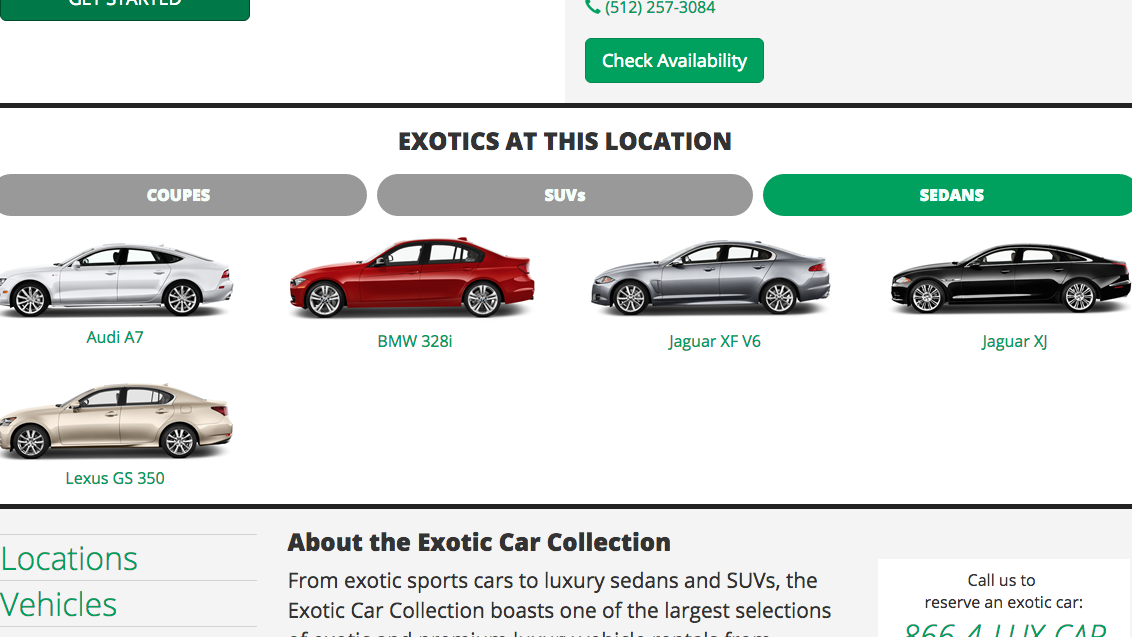A close-up screen capture of a desktop computer screen displays a section of a car dealership webpage. Prominently situated in the upper middle of the image is a phone number, written in green: 512-257-3084. Directly beneath the phone number is a green rectangular button with the white text "Check Availability." Below this button, a thick black horizontal line separates the section header from the rest of the page.

The black text beneath the line reads "Exotics at this location." Following this, there are three horizontally aligned buttons. From left to right, the first button is grayed out and labeled "Coupes," the middle gray button is labeled "SUVs," and the third button is green, with the word "Sedans."

Moving further down, we see five images of cars. The first car in the upper left corner is a silvery Audi A7. To its right is a red BMW 3.8i. The other three cars are not fully visible in this portion of the screen capture. This partial webpage view provides essential information for potential customers interested in exotic cars while showcasing a selection of available models.